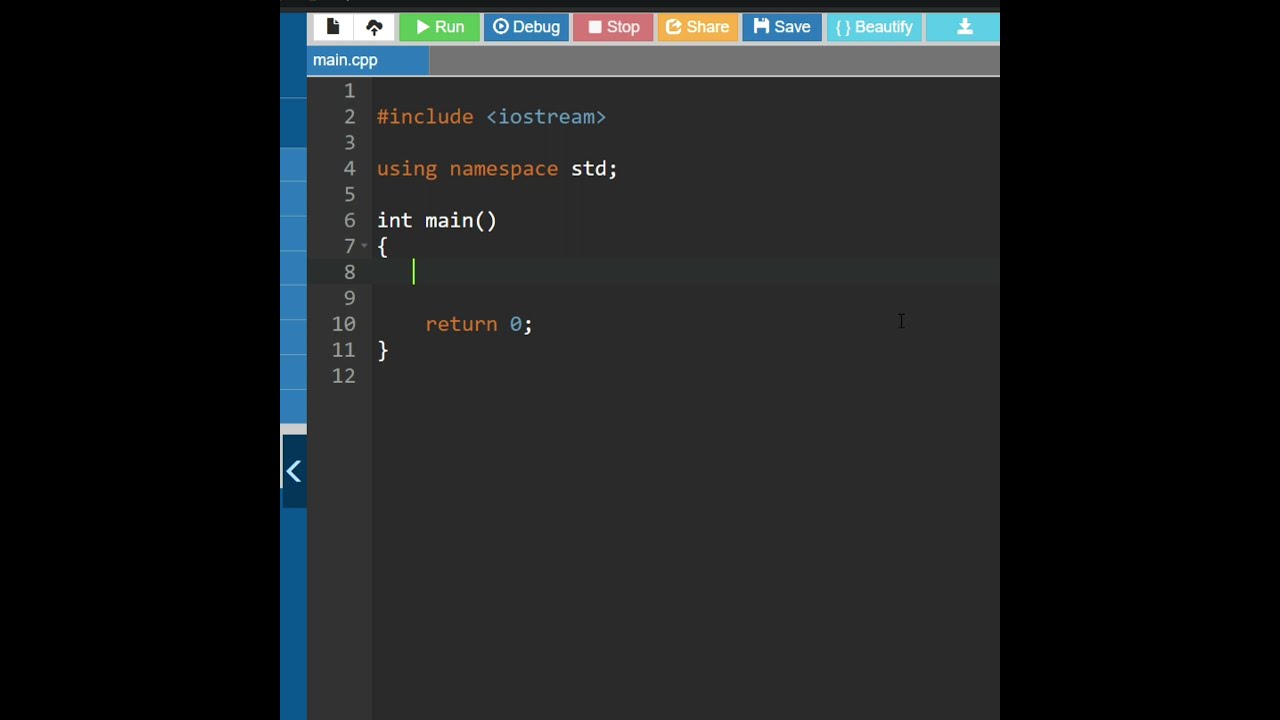The image is a screenshot, likely from an Apple developer's panel or a coding editor, displayed against a plain black background. Central to the image is a dark screen featuring a colorful array of text and icons. Starting from the top, there are button labels for "run," "debug," "stop," "share," "save," and "beautify." These buttons suggest a software development environment. The code in the screenshot includes various programming keywords and syntax such as `#include <iostream>`, `using namespace std;`, along with a function declaration `int main()`. The code is color-coded: keywords and brackets in blue, comments or strings (if present) in green, and operators and symbols in red, yellow, and white. A cursor highlighted in lime green is also visible. On the left side of the screen, line numbers 1 through 12 are displayed in a column. This organized layout of code and tools is indicative of a coding interface designed for app development or script writing.